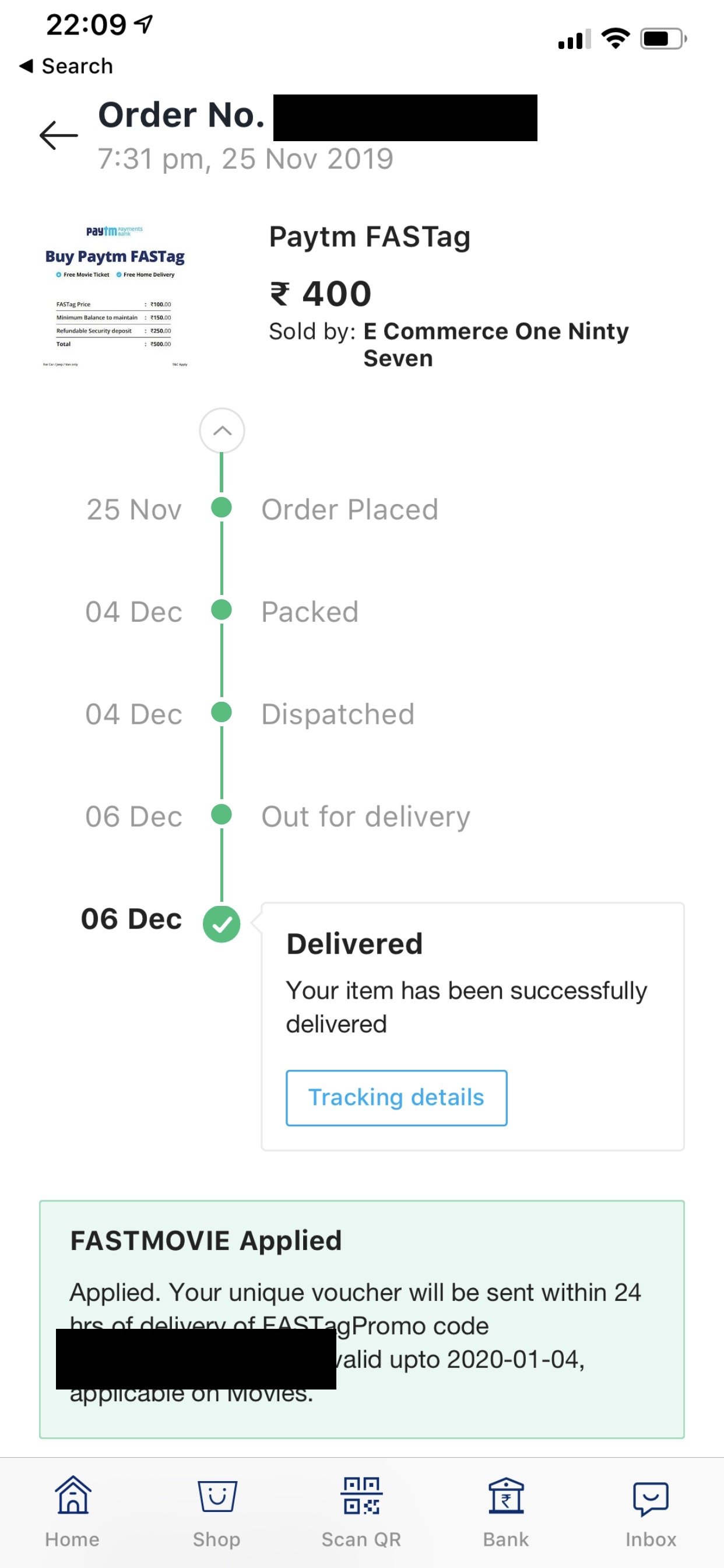This is a detailed screenshot taken on an iPhone device showcasing a completed order on PayTM FastTag. The order, amounting to 400 yen, was placed with the seller ecommerce187 and marked as delivered on the 5th of December. Additional tracking details for the shipment are also visible. A promotional offer, "FastMovie," has been applied, promising that the customer's unique voucher will be sent within 24 hours of delivery. However, the voucher code is partially obscured by a black rectangle at the bottom of the screen. Similarly, the order number at the top of the screenshot has been blocked out with a black rectangle. The order notification indicated that the purchase was confirmed at 7:31 PM on the 25th of November, 2019. Adjacent to the order number, there is a small image serving as proof of notification. The screenshot also reveals that the iPhone's battery is more than half charged and it is connected to WiFi.